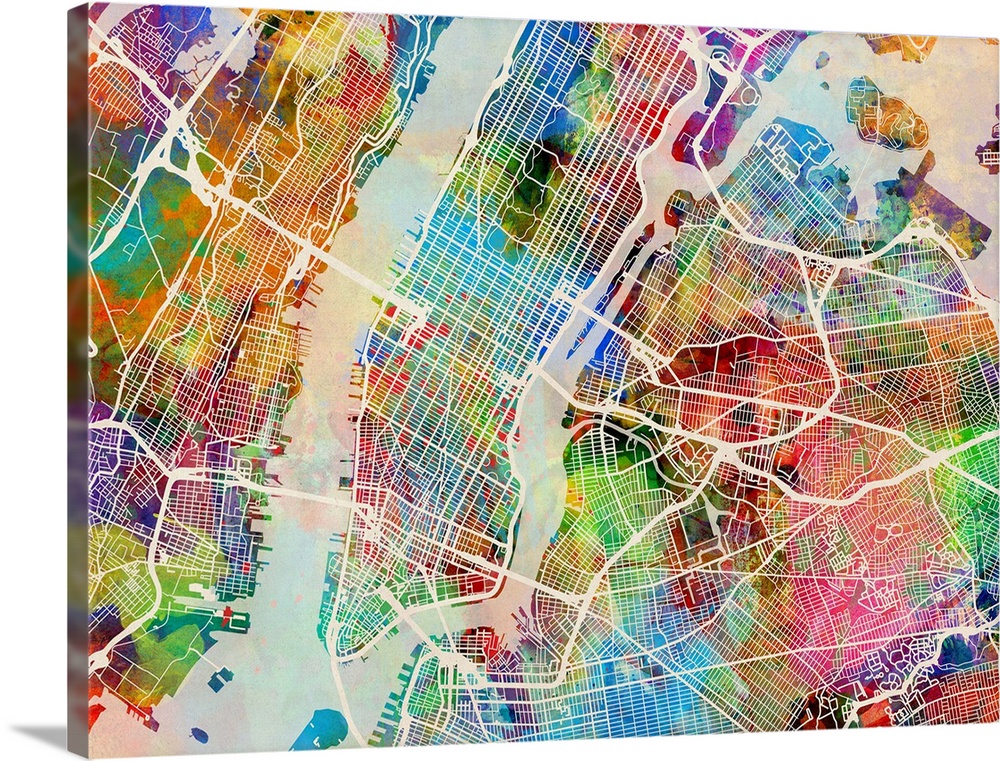The image is a vibrant, multicolored map-like artwork on canvas, viewed slightly from the left to reveal its depth. Dominated by an array of colors reminiscent of a rainbow—greens, blues, reds, oranges, purples, pinks, and multiple shades of green including neon and lime—it portrays an intricate representation of landmasses and waterways. The main features are large white streaks which suggest bridges and roads, potentially spanning gray areas that imply bodies of water. These white streaks bisect checkered and zigzag patterns that might indicate city centers or buildings, despite the absence of a legend. The artwork depicts multiple islands: a large one on the left, another central one with a smaller adjacent landmass below, and the largest on the far right, accompanied by three small flanking islands and another situated between the central and rightmost islands. The complex overlay of translucent white and ivory areas adds depth, hinting at a dense network of rivers, streets, and highways that grids the vibrant landscape. This detailed depiction possibly mirrors a cityscape, like New York, with its bridges, piers, and urban blocks meticulously illustrated.